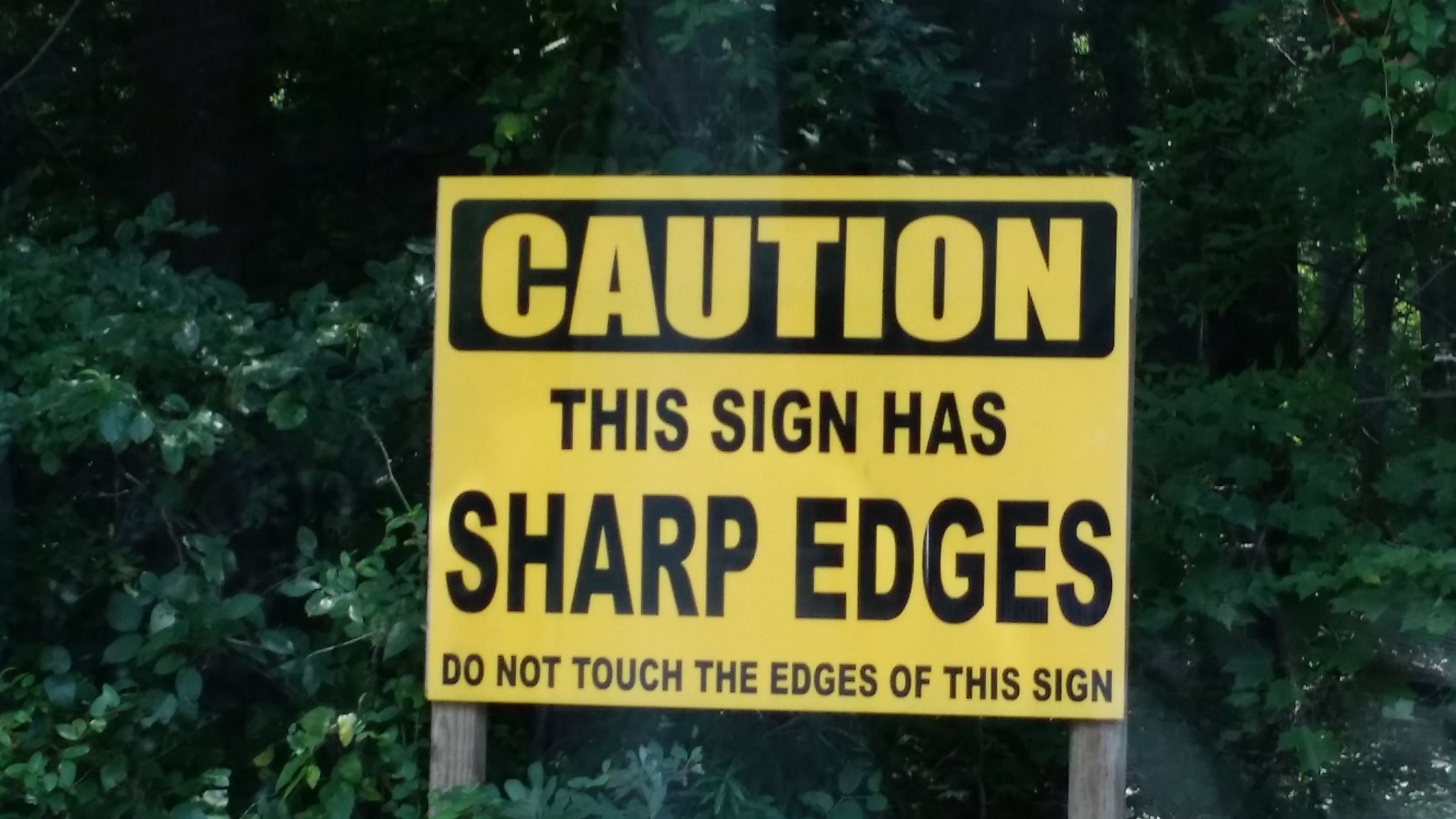In this vibrant outdoor photograph, lush green foliage envelops the surroundings, with an abundance of bushes, plants, and trees creating a dense, verdant backdrop. Amidst this natural splendor, a few scattered rocks can be seen, adding a rustic charm to the scene. Sunlight streams gracefully through the canopy, casting a warm, dappled glow on a notable focal point: a square, yellow sign mounted on two sturdy wooden legs. The sign bears a cautionary message in bold black lettering. The words "CAUTION" and "SHARP EDGES" are prominently displayed in a large font, while a smaller font warns, "Do not touch the edges of this sign." The interplay of light and nature, combined with this humorous yet practical warning, makes for a uniquely captivating image.